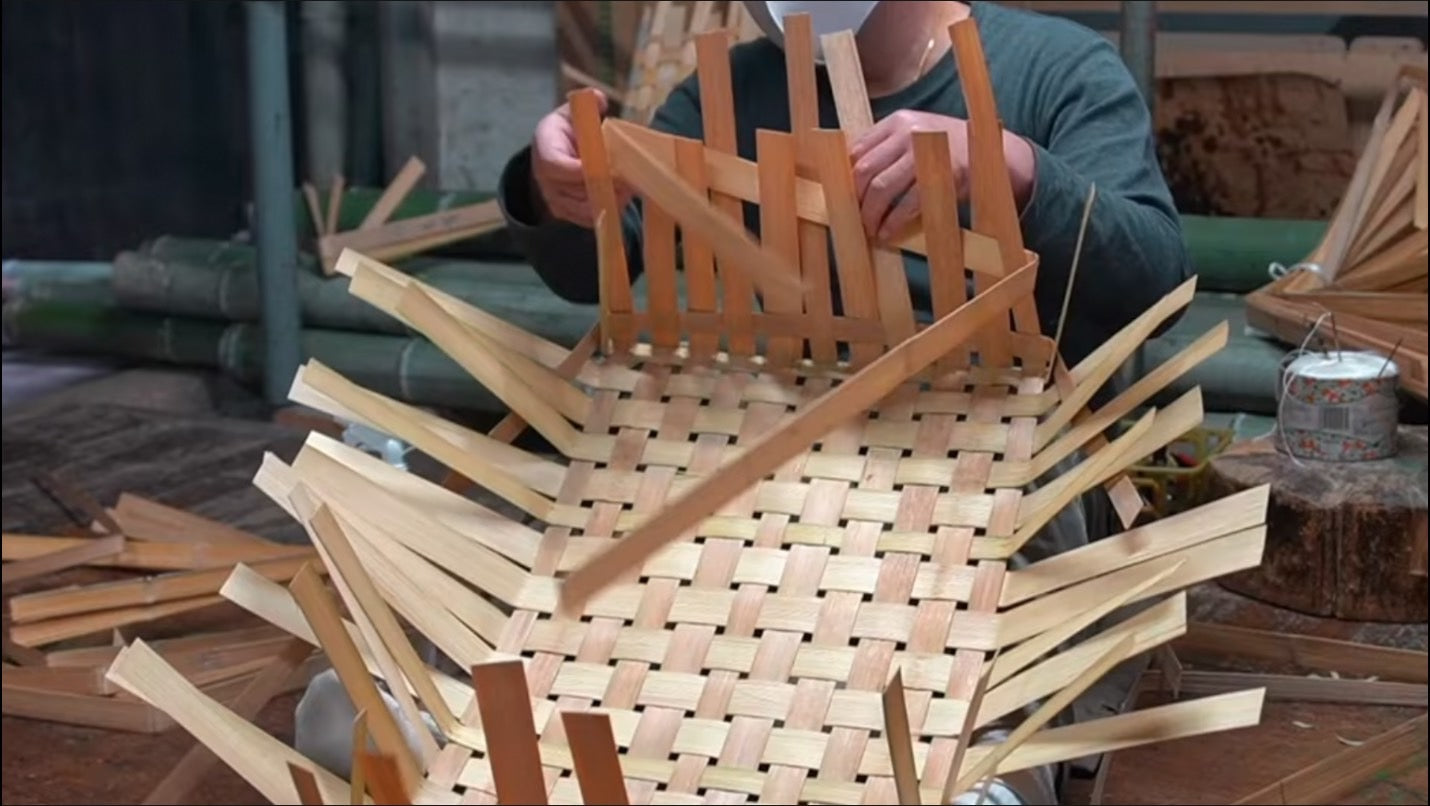In a bustling workshop filled with the scent of fresh wood and the clutter of tools and materials, a craftsman sits on a small stool, weaving an intricate basket. His masked face is partially visible, emphasizing his focused intent on his laborious task. The project appears to be a large woven basket, possibly an Easter basket, with thin, brownish wood strips deftly crisscrossed in a checkerboard pattern. The base of the basket is completely woven, showcasing an expertly crafted foundation, while the sides, with wood slats bent upwards, await further weaving. Strewn around him are various tools and a large spool of white string, along with large needles that aid in securing the weave. The basket sits in his lap, elevated slightly as he manipulates the materials, suggesting a deep dedication to his craft, while the organized chaos of tools and supplies indicates a space dedicated to meticulous workmanship.